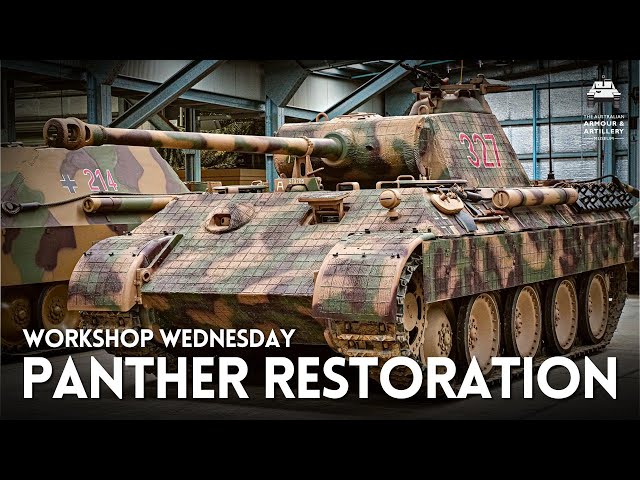The image features a spacious warehouse with light blue steel beams and gray panel walls. At the center and to the right, we see two camouflaged tanks. In the foreground, a fully visible tank with a camouflage pattern of green, light brown, and black displays the number 327 in red on its side. This tank is equipped with a large turret, a cannon, and a machine gun on top, and it has a tan-colored roller wheel structure. Beside it, another tank also camouflaged and marked with the number 214 in red, features additional armor on its top along with a blue cross insignia. Superimposed on the image at the bottom are the words "Workshop Wednesday" and "Panther Restoration" in bold white text. The upper right corner bears the logo and name "The Australian Armour and Artillery Museum," also in white, with the logo depicting a front perspective of a tank. The image is framed by black bars at the top and bottom.